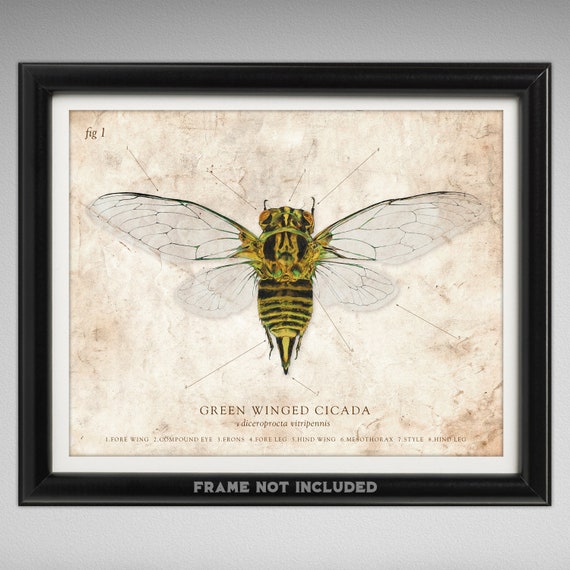The image showcases an intricate, realistic drawing of a green-winged cicada centered on an off-white, creamy-colored background. The cicada, depicted with meticulous detail, features transparent wings with green veins, striking red eyes, and short antennae. Its body displays a pattern of green, black, and faded yellow markings, resembling the color scheme of a bumblebee. Accompanying the artwork is labeled text identifying various anatomical parts like the forewing, compound eye, fronds, foreleg, hind wing, mesothorax, and hind leg, though this text is difficult to read at a glance. This detailed illustration is framed by a white border within a black frame, against a plain gray background. Note that the frame is not included with the purchase of the picture.